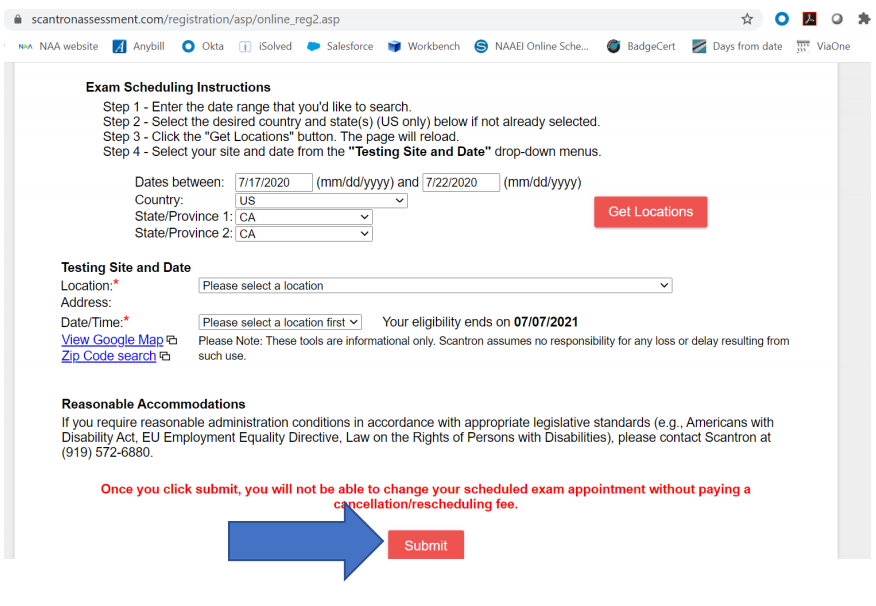A screenshot of a webpage with the URL "scantronassessment.com/registration/ASP/online_REG2.ASP" visible in the address bar. The bookmarks toolbar is populated with several bookmarks labeled: "NAA website," "anybill," "opta," "isolve," "salesforce," "workbench," "NAAEI online," "badge cert," "days from date," and "via one." The body of the webpage outlines an exam scheduling process with detailed instructions as follows:

1. Enter the date range you wish to search.
2. Select the desired country and state (US only), if not already selected.
3. Click the "Get Location" button, causing the page to reload.
4. Choose your preferred site and date from the "My Testing Site and Date" drop-down menus.

A prominent red button labeled "Get Locations" is placed below the instructions, and another red button labeled "Submit" is located at the very bottom of the page. The "Submit" button is highlighted by a large blue arrow pointing directly at it from the left side of the page.